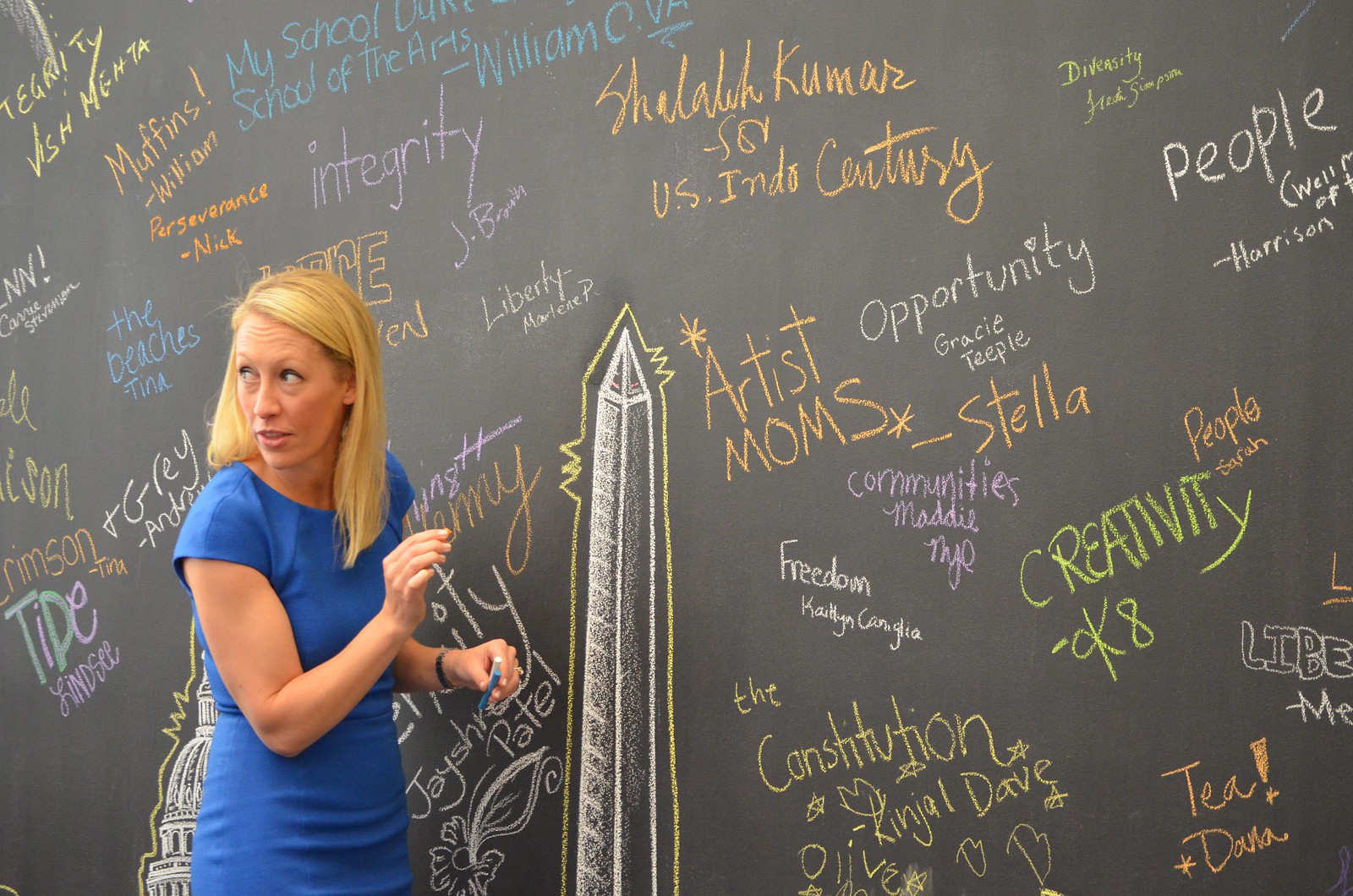In this image, a woman stands left of center in front of a large black chalkboard covered with various writings and drawings in an array of colors, including yellow, green, orange, purple, blue, and white chalk. She is dressed in a blue dress, and her yellow-blonde hair falls to her collarbone. She holds a piece of white chalk and a piece of blue chalk in her hands. The chalkboard behind her features a prominent drawing of the Washington Monument in the center, outlined in yellow. There is also a depiction of the Capitol building behind her. Surrounding these illustrations are numerous cursive and handwritten words and phrases such as "artist moms," "Stella," "the Constitution," "creativity," "integrity," "liberty," "Maddie," "Caitlin," "Dave," "diversity," "U.S.," "Tina," "my school," "Nick," and "William." Additionally, hearts and other doodles adorn the board, contributing to the vibrant and eclectic backdrop. The woman gazes towards the left side of the image, away from the chalkboard, adding a contemplative feel to the scene.